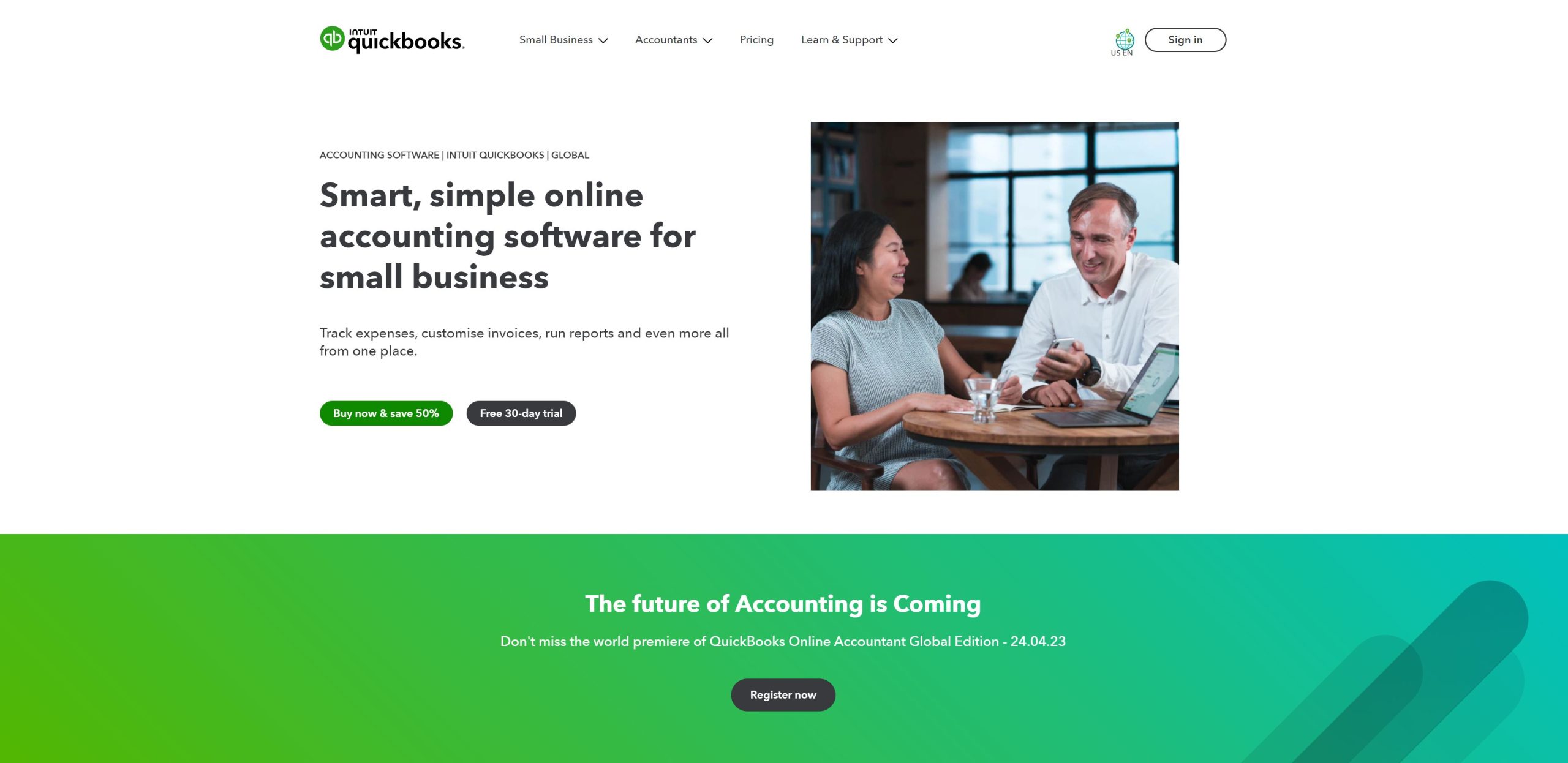This image captures the homepage of the Intuit QuickBooks website. Dominating the top-center area, slightly to the left, is the recognizable green logo featuring the lowercase "qb" letters with stems extending vertically. Adjacent to it, in bold black text, appears the branding "Intuit QuickBooks."

Below this header lies a navigation bar containing multiple dropdown menu options, including "Small Business," "Accountants," "Pricing," and "Learn and Support," each accompanied by a down arrow for further selections. Towards the far right of the navigation bar is a prominent sign-in button shaped like a pill with black text inside.

Directly underneath the logo and navigation options, the tagline "Accounting Software Intuit QuickBooks Global" is displayed in prominent text. Beneath this, another bold message reads "Smart Simple Online Accounting Software for Small Business." This is followed by a succinct description outlining features such as "Track Expenses, Customize Invoices, Run Reports, and even more all from one place."

Further down, two call-to-action buttons are presented: a green button encouraging visitors to "Buy Now and Save 50%" and a gray button offering a "Free 30 Day Trial." Adjacent to these buttons is an image depicting two people in a discussion at a coffee table, symbolizing business collaboration.

At the bottom of the image, a prominent green banner declares "The Future of Accounting is Coming," hinting at forthcoming advancements or updates in the QuickBooks software.